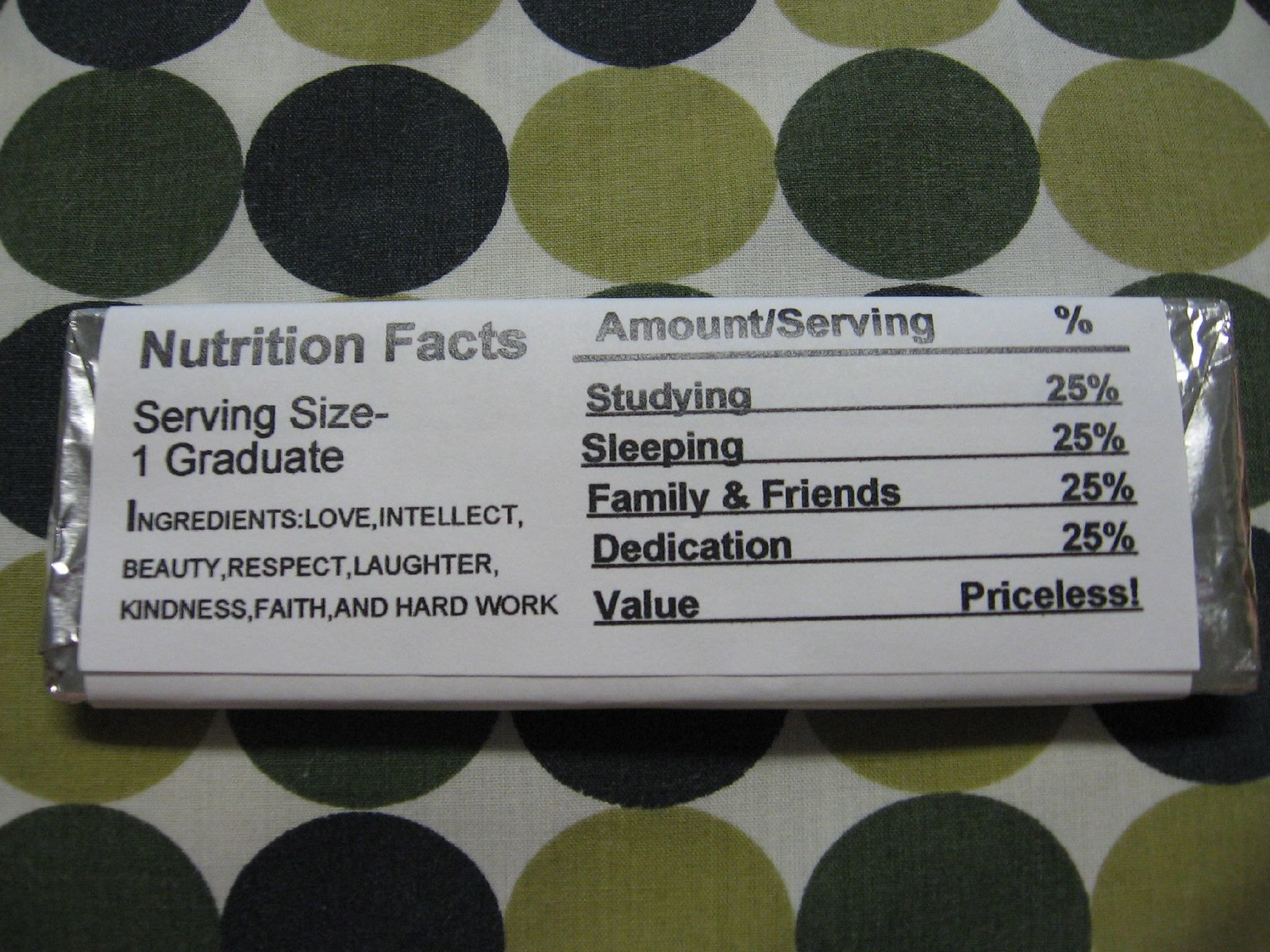The photograph depicts a horizontal image of what appears to be a candy bar wrapped in a white, flexible package sealed in aluminum foil. The wrapper, resembling nutrition facts on a typical food package, whimsically lists the serving size as "One Graduate." The listed ingredients are love, intellect, beauty, respect, laughter, kindness, faith, and hard work. On the right-hand side, the wrapper details the "Amount Per Serving" with percentages: Studying, 25%; Sleeping, 25%; Family and Friends, 25%; Dedication, 25%; and states the value as "Priceless." The candy bar rests on a tablecloth adorned with a 60s-era pattern featuring interconnected dots in varying shades of green, brown, and grayish-green on a white background. The dots are arranged in regularly spaced rows and columns, enhancing the vintage aesthetic of the setting.